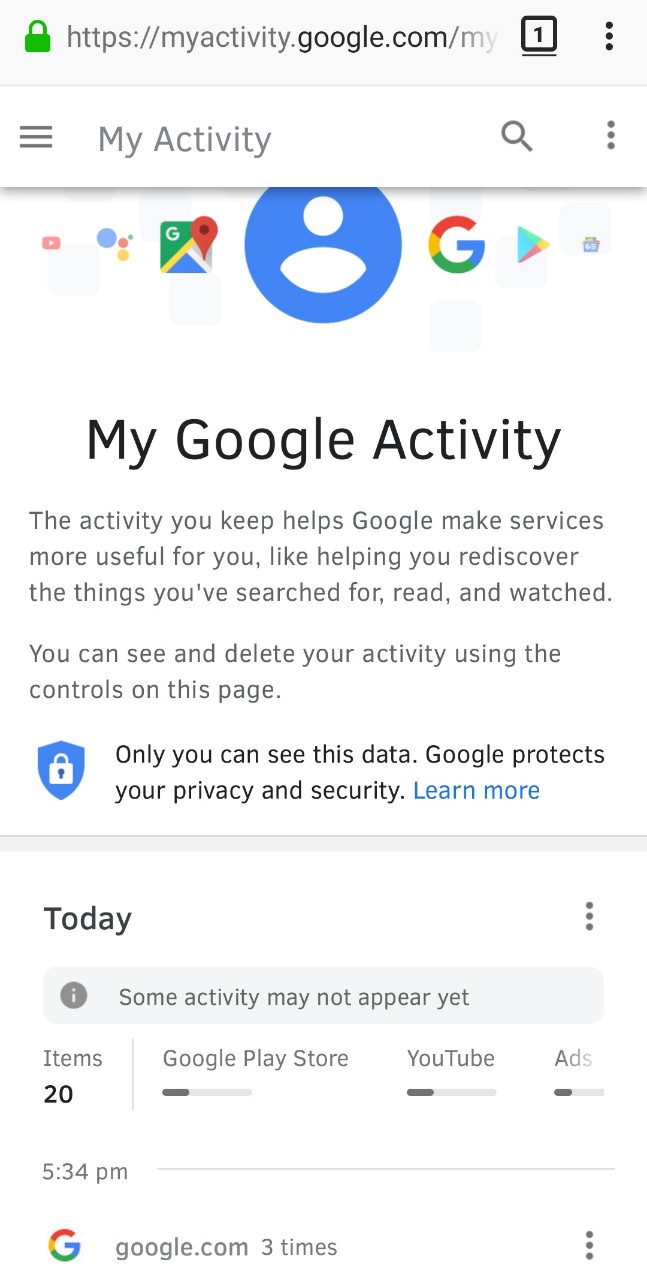The cell phone screenshot displays the Google My Activity page. At the top, the address bar shows a secure connection symbolized by a green lock followed by the URL: "https://myactivity.google.com." To the right of the URL, a notification indicator displays the number "1," and three horizontal dots are present for additional options.

Below the address bar, there is a white navigation strip with a hamburger menu (three horizontal lines) on the left, the title "My Activity" in the center, and a magnifying glass icon (search) along with another set of three horizontal dots on the right.

The main content starts with an array of icons representing Google services such as Google Maps, Messenger, and the Play Store. Below these icons, the text "My Google Activity" is prominently displayed, followed by a message explaining how the activity data stored helps Google improve user experience by making services more useful. This section also mentions that users can view and delete their activity via the controls on the page. A blue shield icon with a lock indicates that only the user has access to this data, with a reassurance about Google's commitment to privacy and security and a "Learn more" link for additional information.

Further down, there's a heading labeled "Today" separated by a gray bar that states, "Some Activity May Not Appear Here." The subsequent section lists recent activity: "20 items" under categories like Google Play Store, YouTube, and "google.com," with timestamps, including one noted at "5:34 PM."